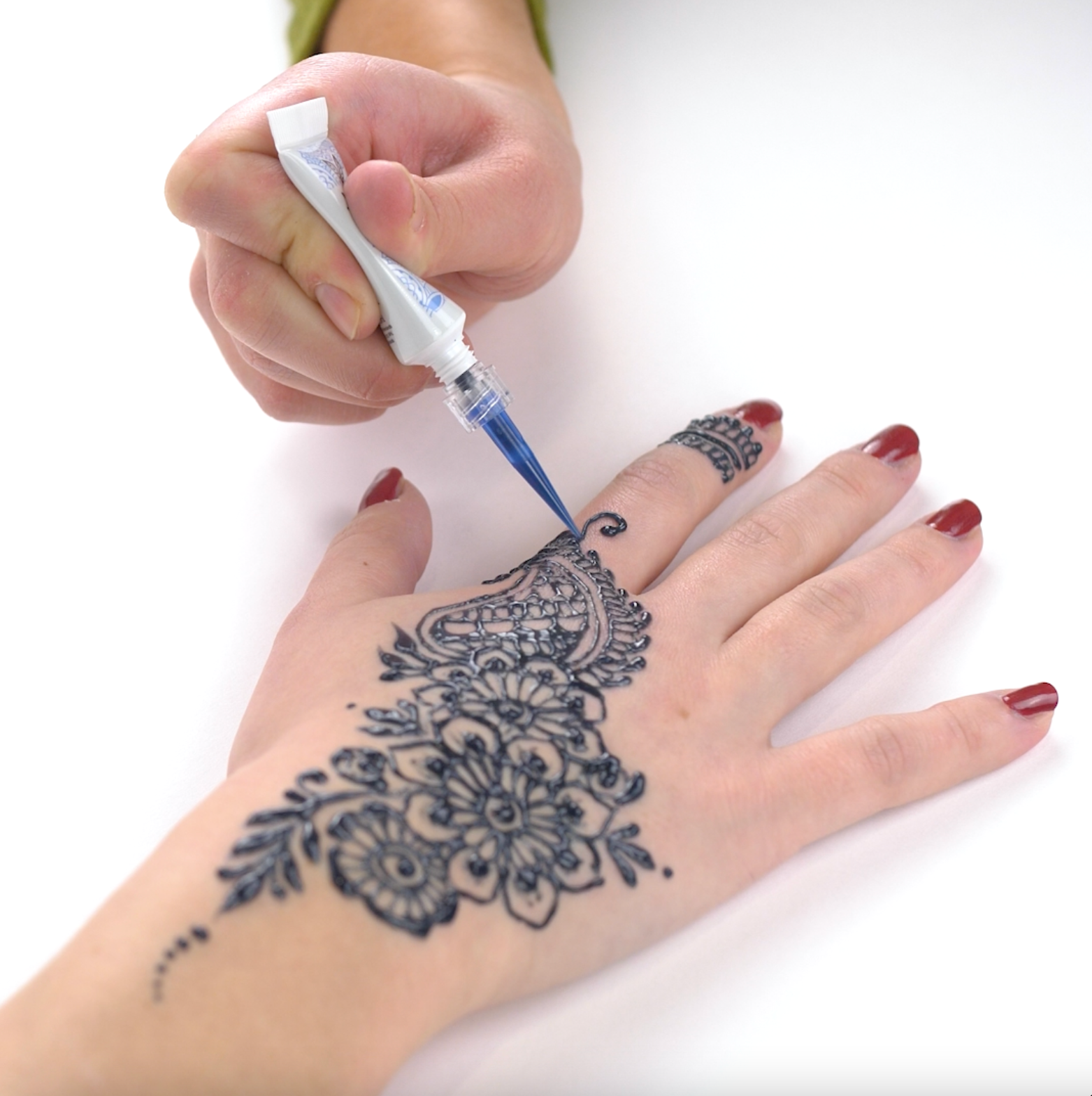This close-up photograph captures a detailed moment of a henna artist at work, applying an intricate, ornate design on another woman's hand. The image features two Caucasian hands: the hand being decorated lies flat against a white table, adorned with dark red, glossy fingernail polish. The henna design, in deep blue ink, beautifully spreads from the wrist to the tip of the index finger, featuring an array of flowers, swirls, leaves, and geometric patterns. The artist, identifiable by her green sleeve visible up to her wrist, holds a white tube with a long, blue-tipped nozzle that dispenses the henna. The paint appears thick and slightly raised, adding texture to the already elaborate pattern. The composition and proximity of the photograph provide a rich, detailed view of the henna application process, highlighting both the fineness of the artist's work and the vivid colors involved.